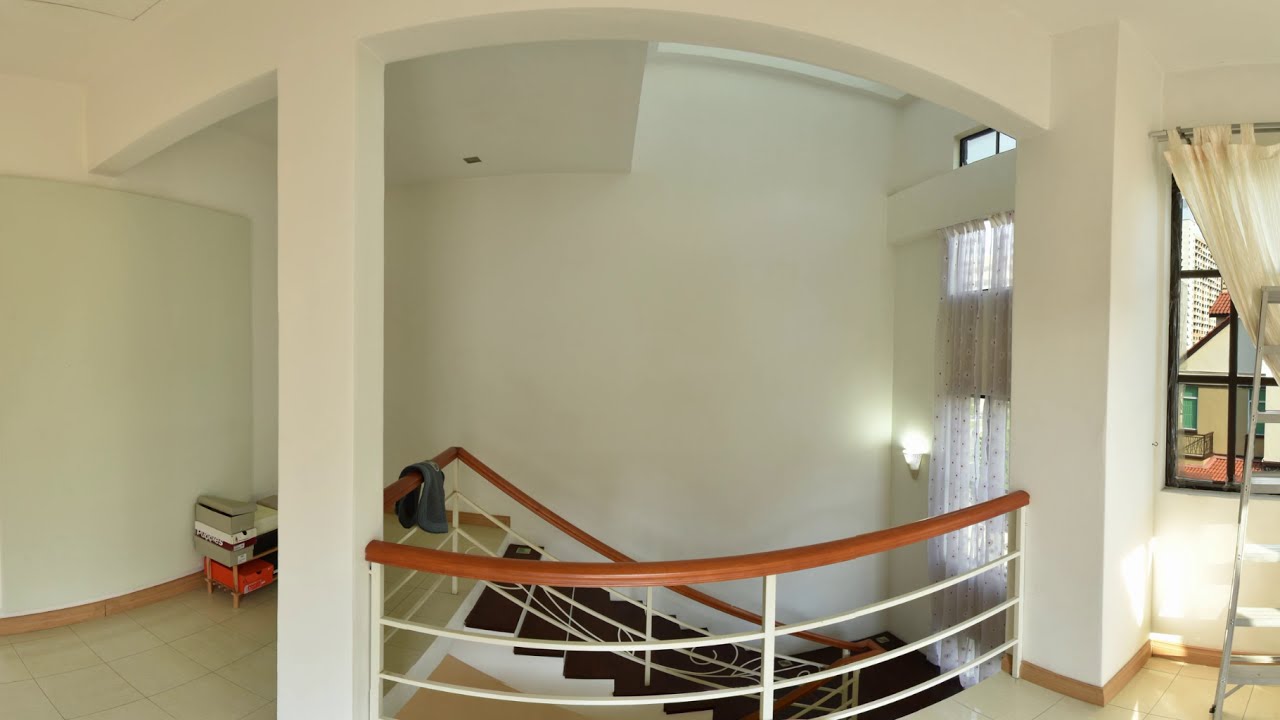The image depicts an interior stairwell of a house with a distinctive and elegant design. The staircase features a combination of white steps with black tops, transitioning down to a tiled landing area. The stair railings are composed of sleek metal bars, crowned with a rich, tan-brown wooden banister. The stairs lead from mid-level to another, with a downward set beneath them. The ceiling above the staircase curves gracefully, likely enhancing the acoustics of the space. A large vertical window, framed in black, adorns the wall adjacent to the staircase, draped with white sheer curtains. Near this window, a silver ladder is positioned, suggesting ongoing construction or cleaning. Additionally, there is sconce lighting ascending the stairwell and a small light fixture beside the window. At the top of the stairs, a small trolley holds various colored shoe boxes, adding a touch of practicality to the stylish setting. The floor is laid with cream-colored square tiles, and the interior walls are painted white, contributing to the room's bright and airy atmosphere.